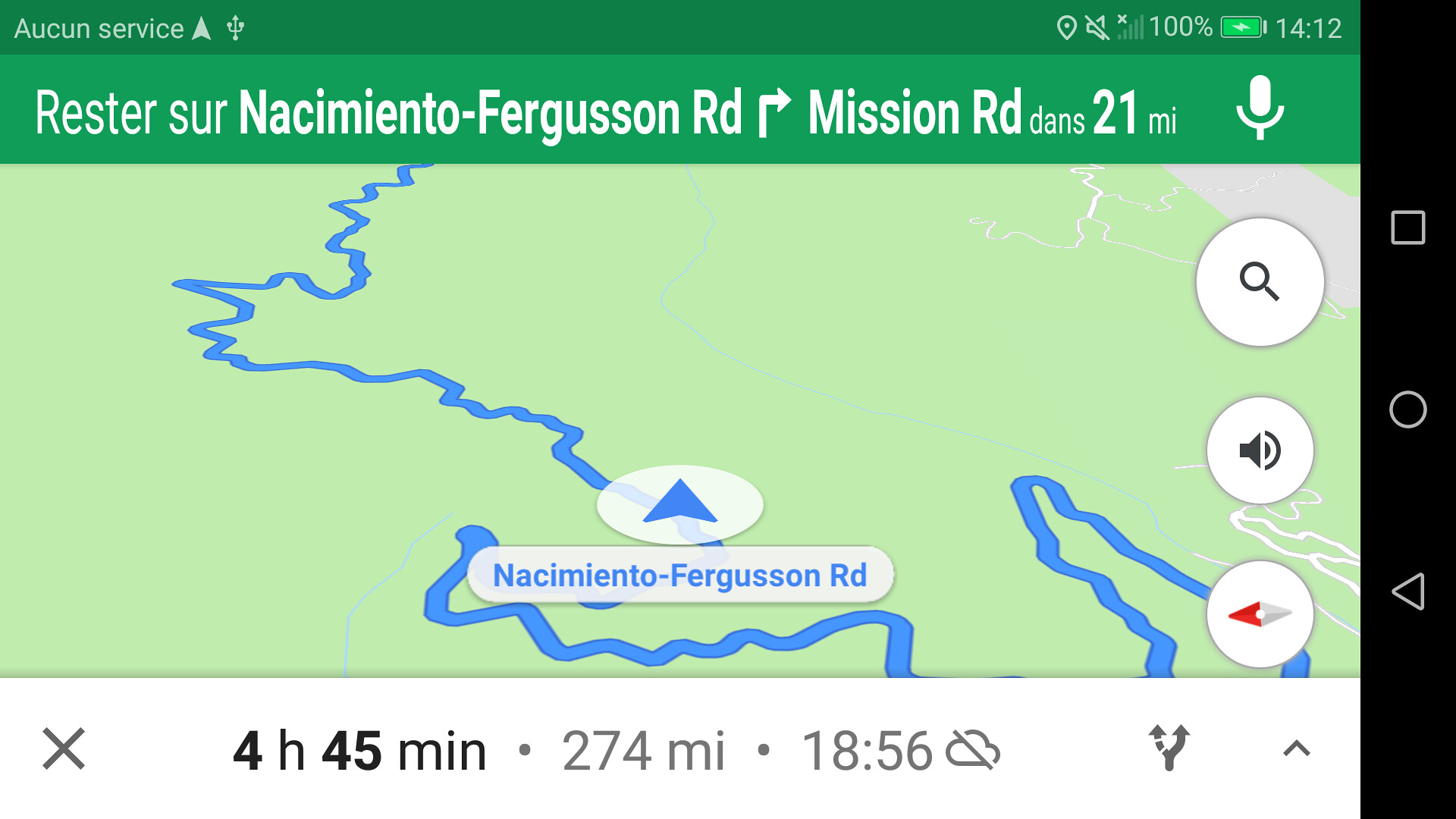This image depicts a detailed screenshot of a Google Maps navigation app displayed on a cellular phone held in a horizontal orientation. The top section of the screen shows various icons, including a triangle, Bluetooth, location, silent mode, signal strength, a fully charged battery (100%), and the current time, 14:12. The main part of the screen reveals a map with a prominent blue winding path, indicating the user's route, marked by a blue arrow within a blue triangle inside a white circle, symbolizing the traveler's current position. Just beneath the top icons, the map shows directions stating "Nacimiento-Ferguson Road" and a future turn, specifying "turn right on Mission Road." Additional features on the screen include a search icon, voice command icon, and compass icon situated on the sides. At the bottom, directions note the journey duration as 4 hours and 45 minutes, covering a distance of 277 miles, with textual instructions also in French, indicating "Rester sur Nacimiento-Ferguson Road" (Stay on Nacimiento-Ferguson Road) and a voiced prompt for the upcoming right turn in 21 miles. The estimated arrival time is displayed as 18:56.